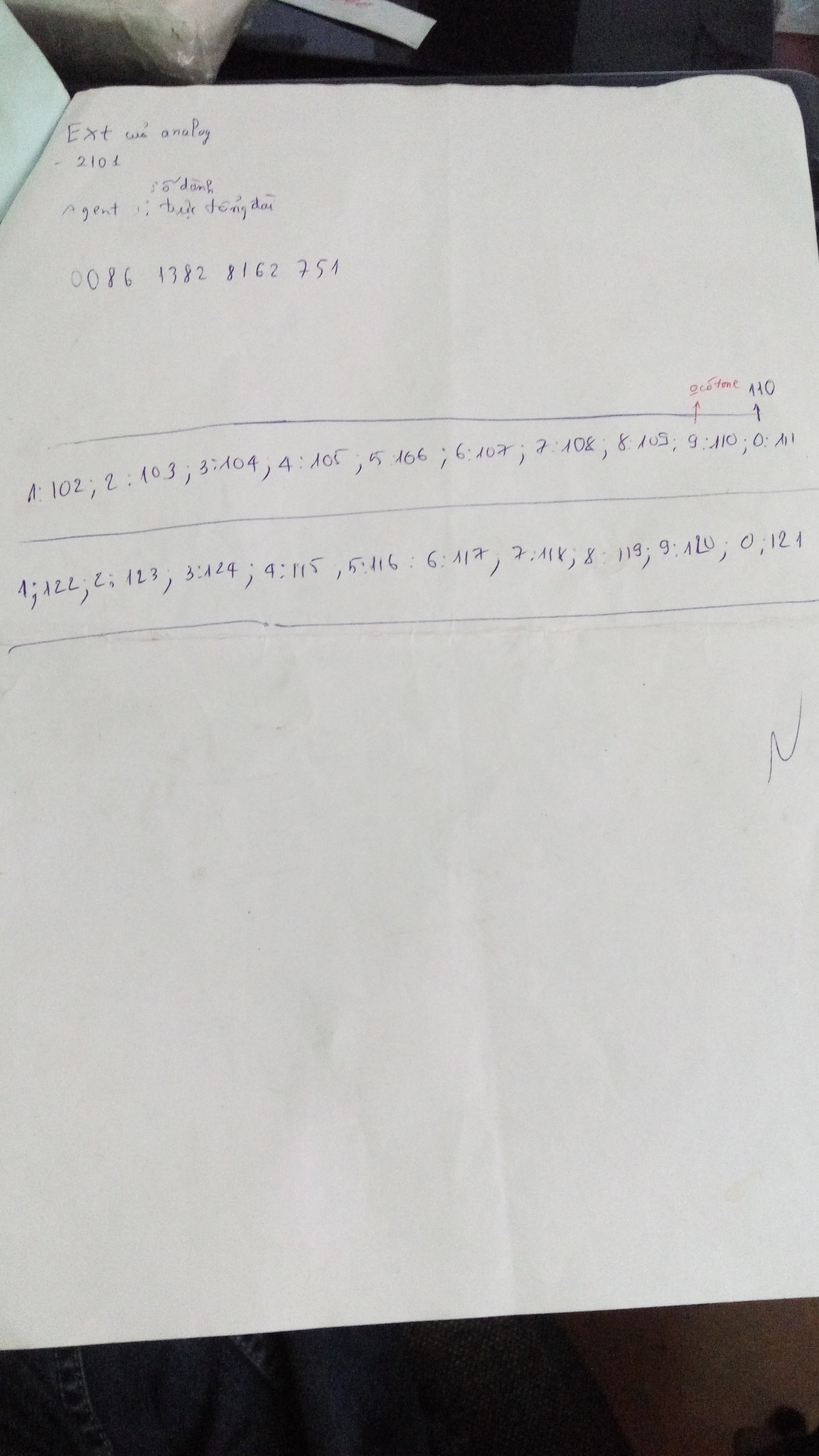In this realistic photograph, the primary focus is a paper that appears to be stapled to another sheet or perhaps bound within a book, making it difficult to distinguish the exact configuration. On the left side, a smaller white page is visible, indicating that the main paper is attached to something larger. Surrounding the page, the background reveals a person's lap, dressed in jeans, suggesting they are holding the notebook. Above this, the background is blurred, showing various indistinct objects.

The notebook or paper displayed is predominantly blank, featuring no lines. At the top left corner, the word "EXTAMANALY" is prominently written, with the number "2101" in smaller text below it. Unreadable smaller text follows beneath "2101." Further down the page, a sequence of numbers, "008613828162751," is shown. Below this series, a horizontal line separates it from a list of numbers: "102, 103, 104, 105, 106, 107, 108, 109, and 110," with another "110" notably marked to the right and underlined. Additional horizontal lines demarcate these sections, punctuating the otherwise stark, blank page.